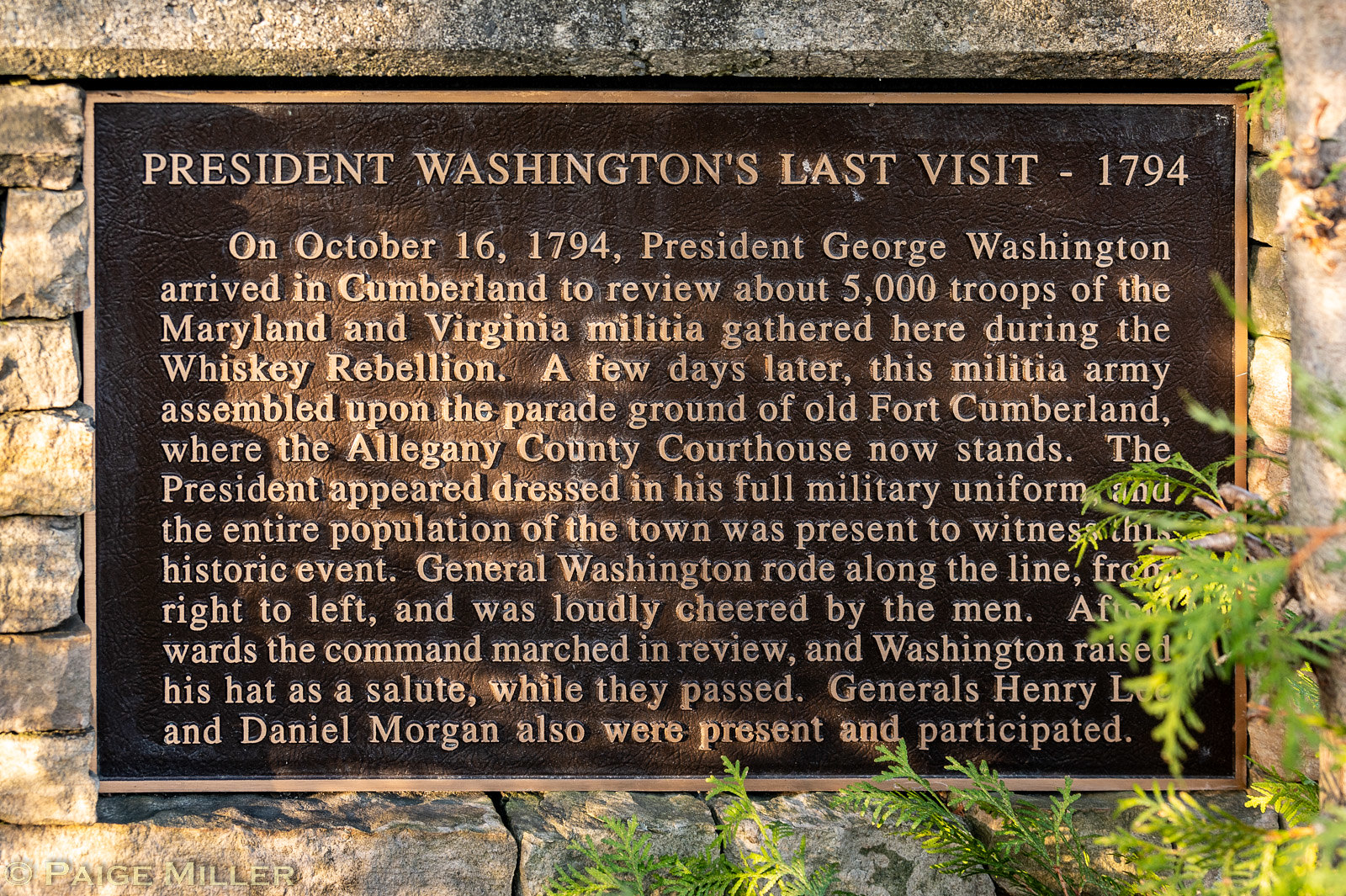The image depicts a historical stone monument surrounded by lush greenery in one corner. Embedded in the stone wall is a black plaque with gold text. The plaque commemorates President George Washington's last visit in 1794. It details how, on October 16, 1794, President Washington arrived in Cumberland to review approximately 5,000 troops of the Maryland and Virginia militia gathered there during the Whiskey Rebellion. A few days later, the militia assembled on the parade ground of Old Fort Cumberland, now the site of the Allegheny County Courthouse. President Washington, dressed in full military uniform, was greeted by the town's entire population. He rode along the line of troops from right to left, receiving loud cheers from the men. As the command marched in review, Washington raised his hat in salute. Generals Henry Lee and Daniel Morgan were also present and participated in the event.